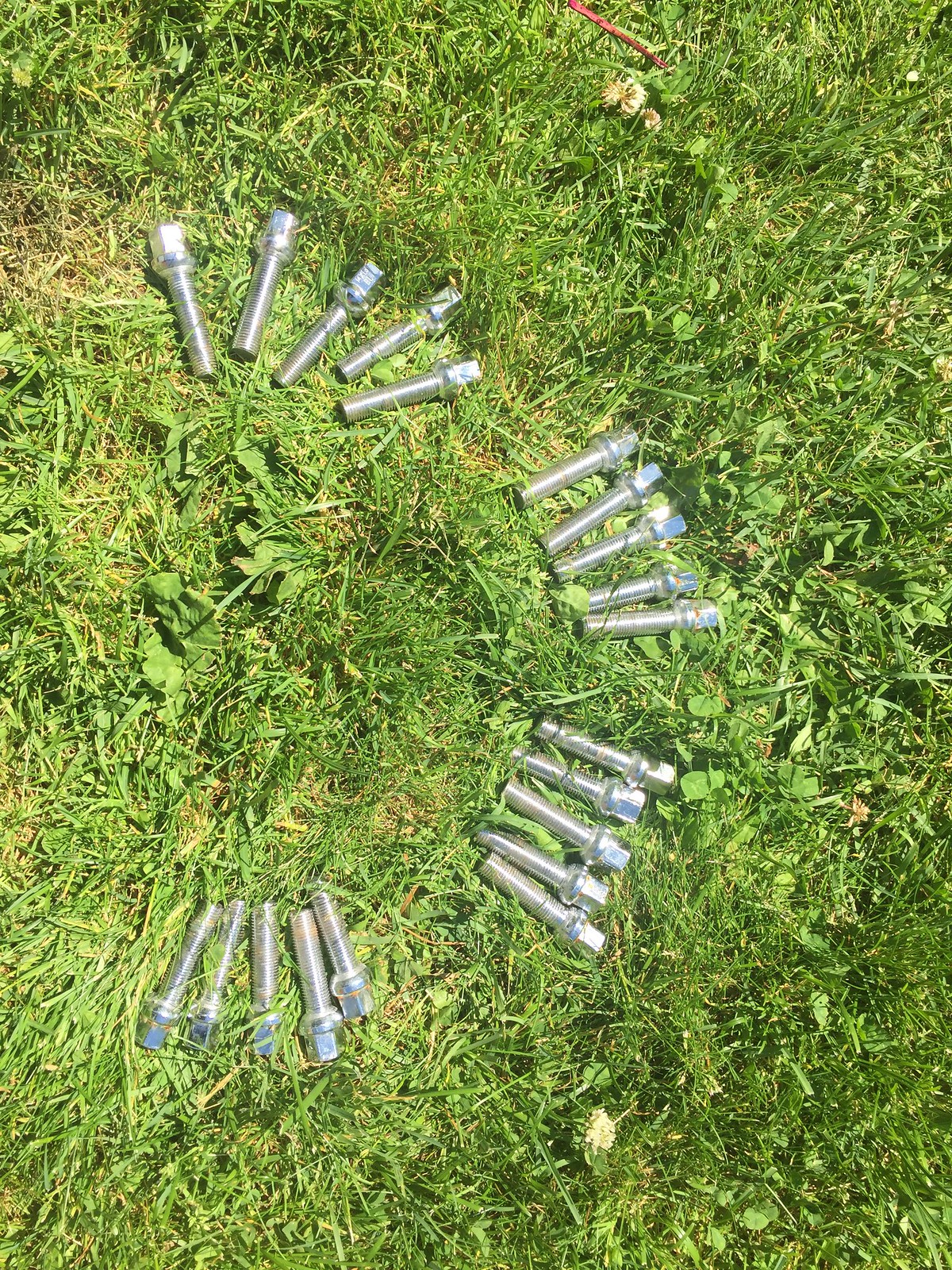This outdoor photograph, taken on a sunny day, captures a grassy lawn featuring short, healthy green grass interspersed with small clover leaves and a few weeds. In the upper right corner of the image, there is a small piece of red paper or plastic. The main focus of the photo is the neatly arranged groups of bolts lying on the grass. There are four groups, each containing five identical stainless steel bolts, aligning in a semi-circular, half-moon pattern. Each bolt is silver in color, with a large hexagonal or octagonal head, a washer or flange below it, and a long threaded area extending from there. The bolts are positioned with their bottom pieces pointing towards the left side of the image.